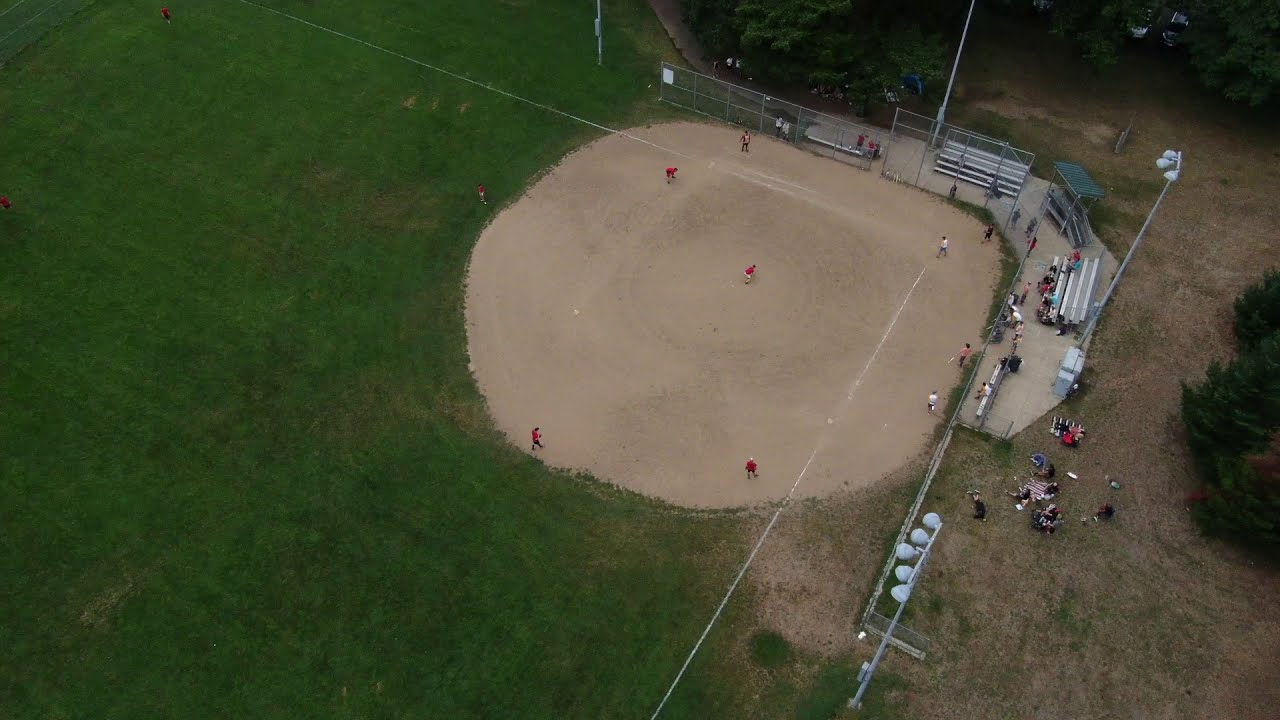This detailed drone image, captured in a landscape orientation and in color, depicts a baseball game in progress from a high altitude. The scene centers around a well-defined baseball field, featuring a brown dirt infield and a lush green grassy outfield. The aerial perspective allows visibility of the specific player positions: an individual at home plate, a pitcher on the mound, and additional players near each base and scattered in the outfield. The teams are distinguishable by their uniforms, with one team wearing white jerseys and black pants and the opposing team in red jerseys with white pants.

The image also reveals the surrounding environment of the game. The baseball field is nestled in a wooded area, with dark green trees framing the scene, particularly noticeable to the right and upper sections of the photograph. Around the field, concrete walkways connect to a main sidewalk, likely leading towards the exit or a parking area. Spectators fill the bleachers behind the fence, keenly watching the game, while others are seated on picnic blankets or in folding chairs, enjoying the match from a slightly more relaxed vantage point. Lighting structures positioned around the field suggest that games can be played after dark. Despite the overcast lighting, the colors remain clear, contributing to the realism and representational style of this drone photograph.